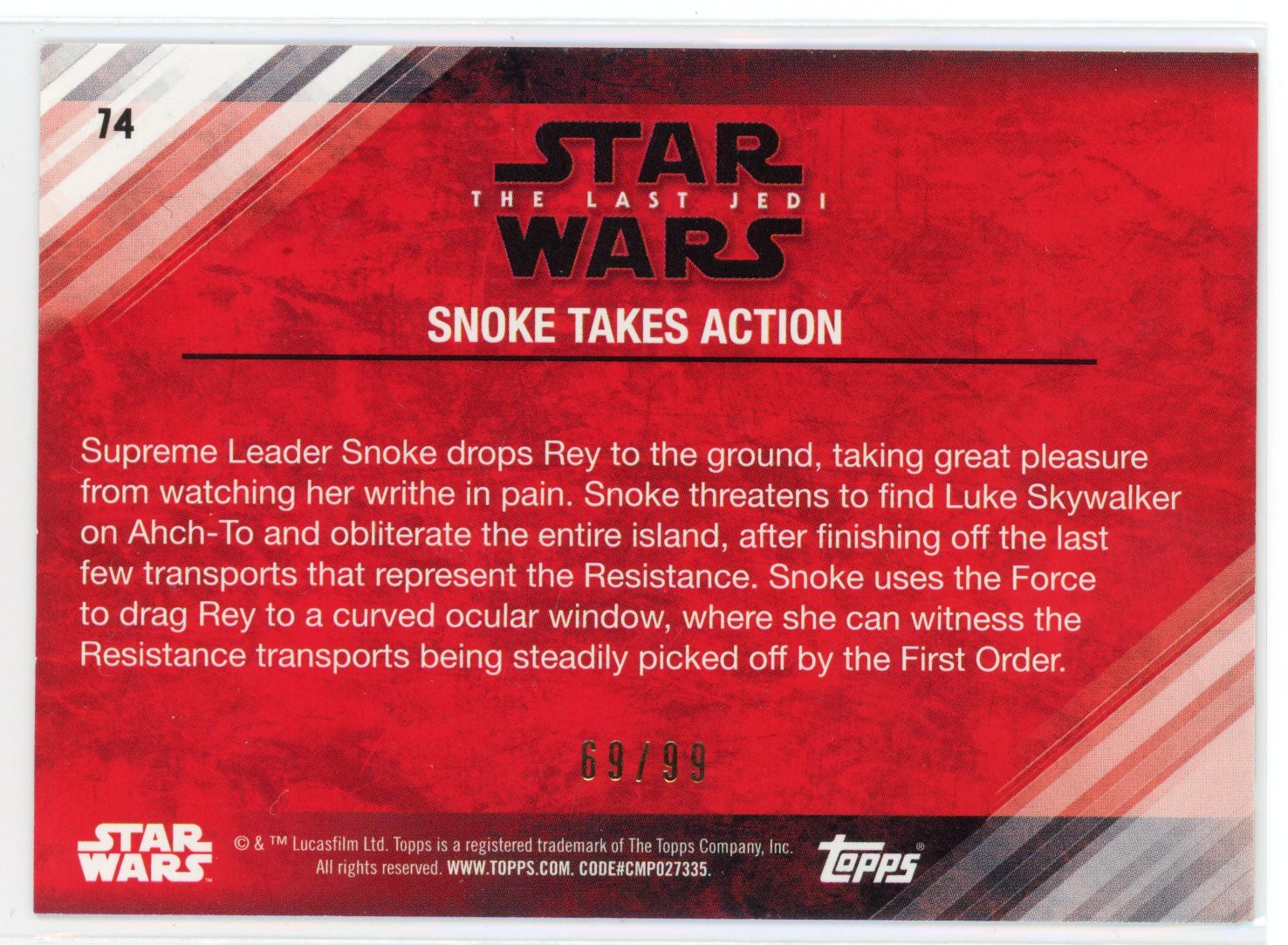This image shows a detailed scan of a collectible TOPS trading card from the Star Wars series, specifically themed around "The Last Jedi." The card features a vibrant red background with black accents, giving it a semi-metallic or velveteen appearance. Centered at the top is the recognizable Star Wars logo in black, with "The Last Jedi" in white text nestled between "Star" and "Wars." Just below this, in all-white capital letters, it states "Snoke Takes Action." A thin black line separates the title from a descriptive paragraph below. 

The paragraph narrates a tense scene where Supreme Leader Snoke drops Rey to the ground, savoring her pain. He then threatens to obliterate Luke Skywalker’s location on the island Ahch-To after destroying the last few Resistance transports. Using the Force, Snoke drags Rey to a curved ocular window to make her witness the First Order picking off the Resistance transports one by one. 

Beneath this narrative, stamped in gold lettering, is "69/99," indicating this card is the 69th out of a limited edition of 99. In the upper left corner, the number "74" is printed in black. At the very bottom, there is a bar with the Star Wars logo, trademark information, and the TOPS logo. Additionally, the inclusion of URLs and trademark details anchors its authenticity. The card, shown inside a plastic cover for protection, is a striking piece of graphic design and illustration, highly detailed and crafted for collectors.